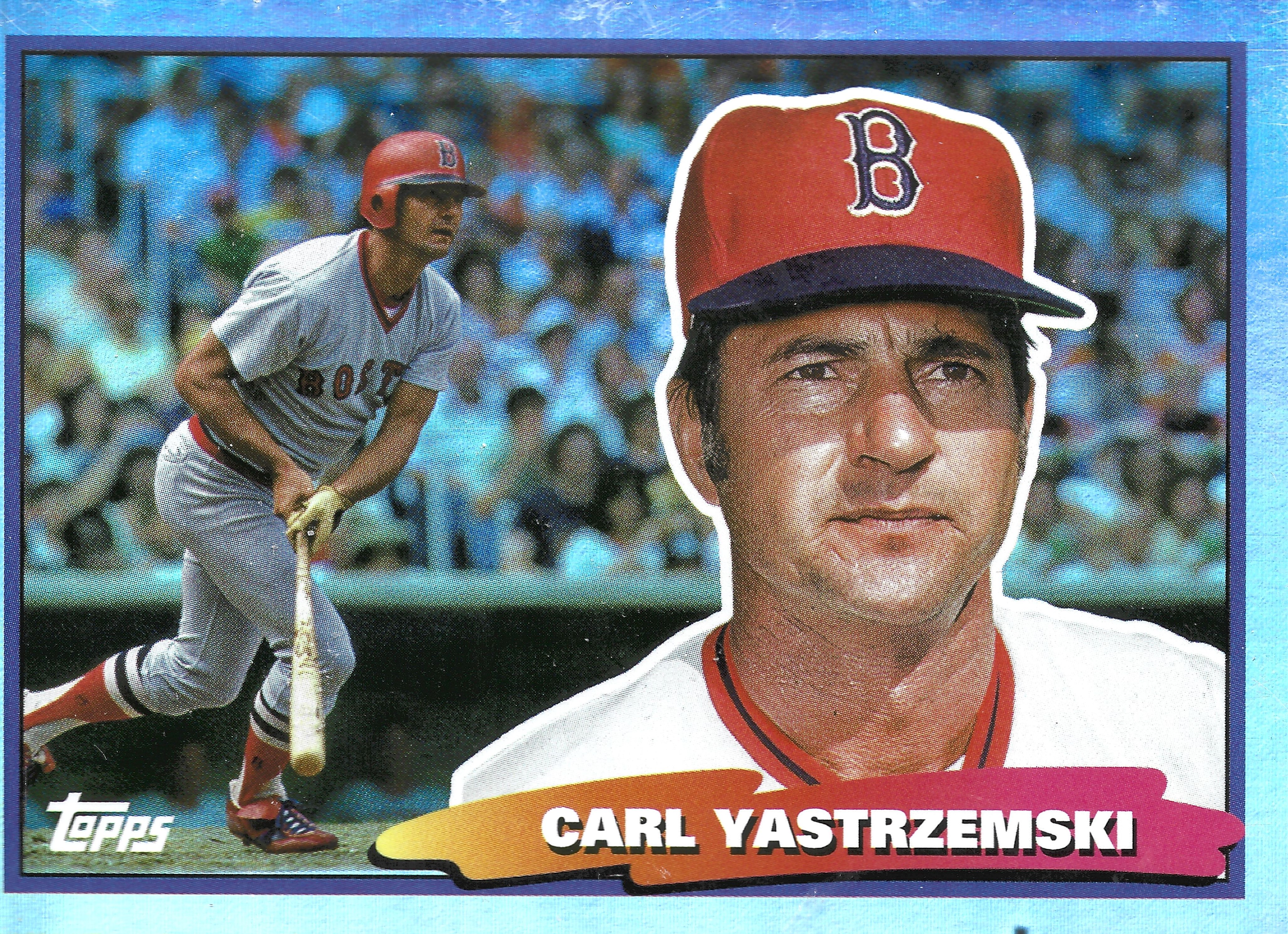The image features a baseball card, identifiable by the small, bold white "TOPPS" logo located in the bottom left corner. Dominating the right side of the card is a head-and-shoulders photograph of Carl Yastrzemski, decked out in his Boston Red Sox uniform, with a baseball cap that has a blue brim and a red top, featuring a blue "B" emblem. His name, "Carl Yastrzemski," is inscribed in a vibrant mix of orange and pink paint-splash text near the bottom right of the card. The left side of the card showcases an action shot of Yastrzemski clad in his white uniform, holding a baseball bat as if he has just hit the ball and is about to run to first base. The background behind both images is filled with slightly out-of-focus baseball fans seated in the stadium stands, adding depth and context to the overall scene.